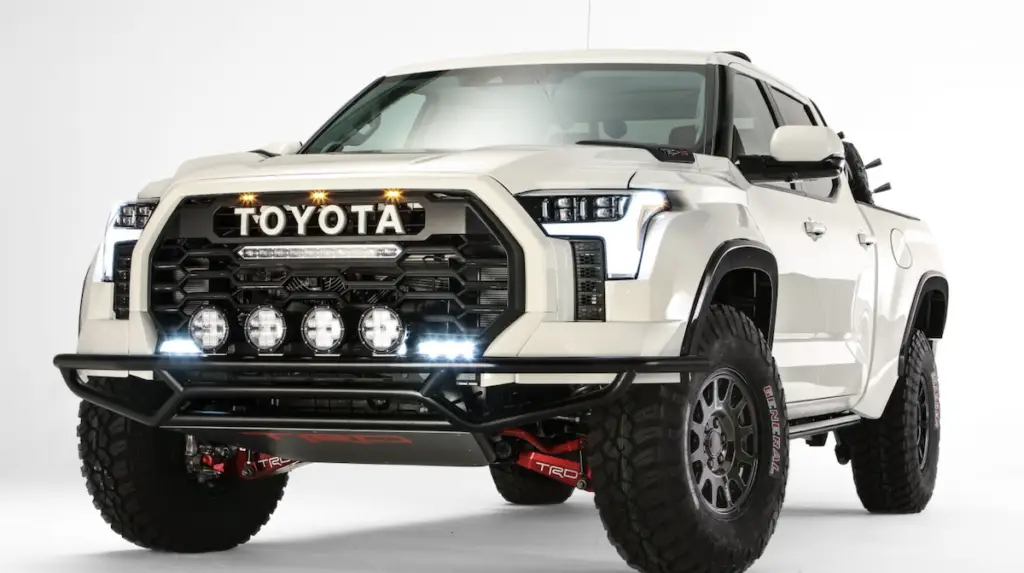This image features a pristine, brand-new Toyota four-door truck set against a plain white background. The truck, which has an ivory white exterior, faces forward, showcasing a prominent black grille with "Toyota" emblazoned clearly across the top. It sports a robust metal bumper and an undercarriage skid plate, highlighting its off-road capabilities. The truck's front is equipped with four round lights at the bottom of the grille, which appear to be illuminated, flanked by rectangular LED lights on both sides, also lit, adding to its aggressive stance. The vehicle stands on large black tires, and it's outlined by a shadow beneath, enhancing the overall sharp and brand-new look. The truck’s two side mirrors and door handles are visible, indicating its four-door configuration, and something indistinct can be seen in the truck bed, along with black elements sticking out. Additionally, two red components are visible underneath the tires, completing the detailed and striking appearance of this off-road-ready Toyota.